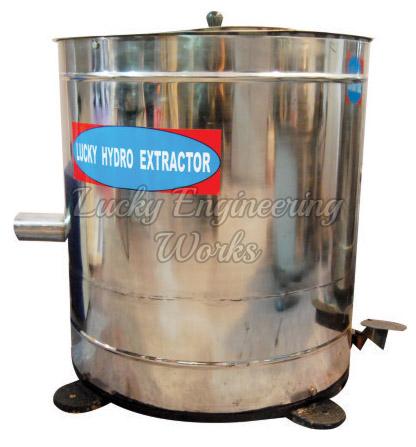The image depicts a large, stainless steel tank labeled "Lucky Hydro Extractor" placed against a plain and completely bare white background. The tank features a lid with a grab knob at the top, a side spigot, and flat legs designed for stable placement, possibly to be bolted to the ground. Additionally, there is a handle on the left side, which may serve mounting purposes. Overlaying the image in the foreground are transparent white letters stating "Lucky Engineering Works," adding to the impression that this is a product page from an engineering website.